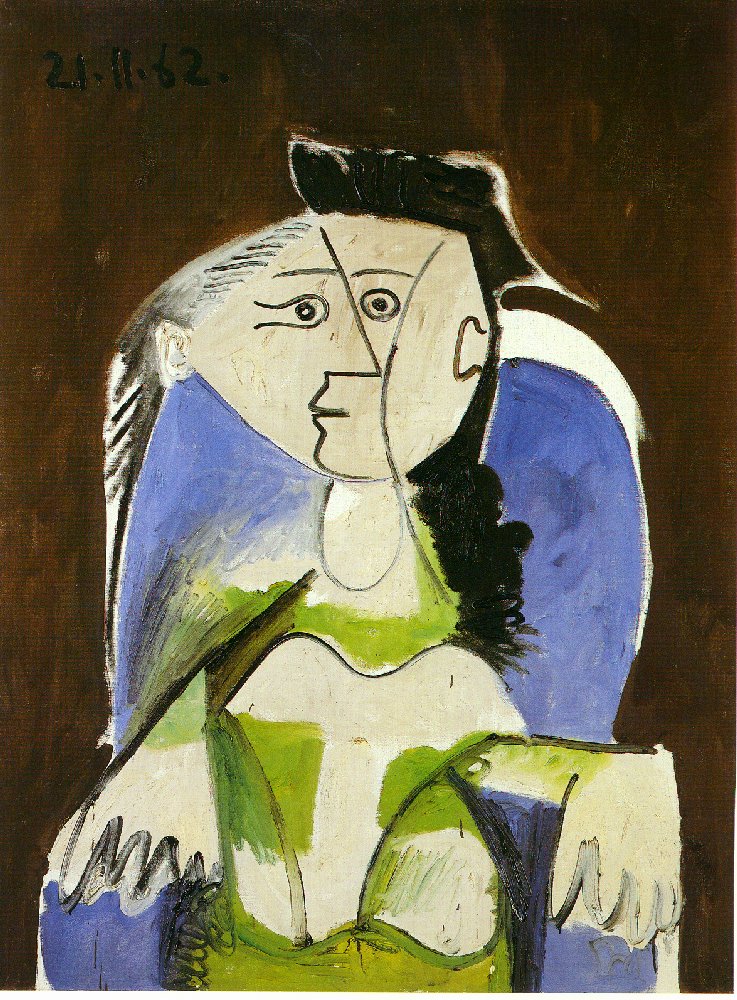This abstract and cubist-style painting features a central figure with a face divided into two distinct halves, reminiscent of Picasso's work. The left side of the face has a sideways eye and slicked back, long black hair, while the right side features a triangle nose and wavy, curly dark brown hair. The background of the painting is a dark, smudged brown, and there are inscrutable black numbers at the top left, potentially reading "25-11-62" or "21-11-62". The figure, combining attributes of a woman, appears to be seated in a blue, abstract easy chair with a white top. She has pale skin and is dressed in a bright, lime-green dress, with her arms outstretched and resting on the chair's armrests. The intricate depiction of her face and body parts, seemingly fragmented and multi-directional, adds to the complexity and abstract nature of the artwork, creating an almost disorienting visual effect.